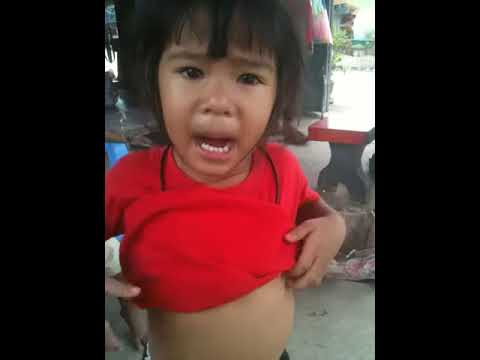The image is a vertical, close-up shot of a young Asian child, possibly between three to five years old. The picture is bordered in black on the left and right sides while the top is without borders, making it taller than it is wide. We appear to be outdoors on a cement patio floor. The child has light to medium brown skin, straight black hair styled with bangs, and dark eyes. The child is looking slightly to the right, with an open mouth showing the tongue and lower teeth, giving an expression of surprise or speaking. The child is wearing a bright red short-sleeved t-shirt adorned with colorful graphics, including a yellow banner with red lettering that spells "BIG" and the number 28. A black string necklace with a circular pendant also adorns the child's neck. In the background, there is a concrete bench on the right side and an open doorway in the upper right-hand corner.